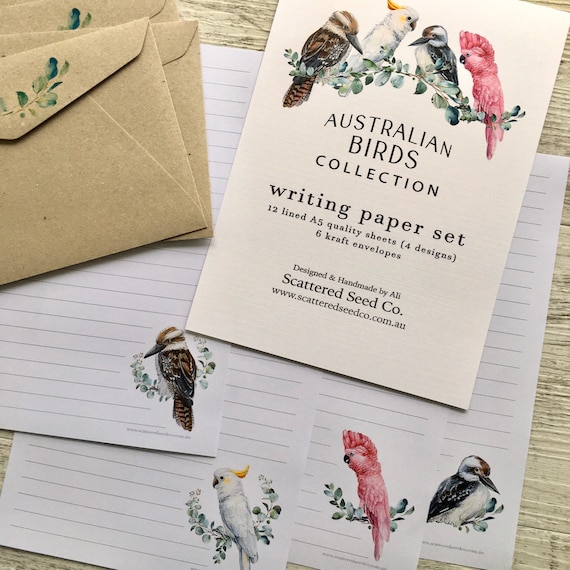The image showcases a meticulously arranged writing paper set named the "Australian Birds Collection." Central to the image is an elegantly designed card introducing the set, adorned with delicate illustrations of various birds like the kookaburra, parrot, and cockatoo. The card reads: "Writing Paper Set - 12 lined A5 quality sheets (4 designs), 6 craft envelopes. Designed and handmade by Allie, www.scatteredseedco.com.au". Surrounding this central card are six brown craft envelopes, each decorated with subtle leaf motifs. Behind and beneath the card lie stacks of lined notepaper, each sheet featuring charming bird illustrations in the corners. The primary colors of the birds include shades of brown, white, red, and black, adding a vibrant yet natural touch to the set. The overall presentation, set against a wooden table, evokes a nostalgic and artisanal feel, highlighting the handcrafted nature of the product.